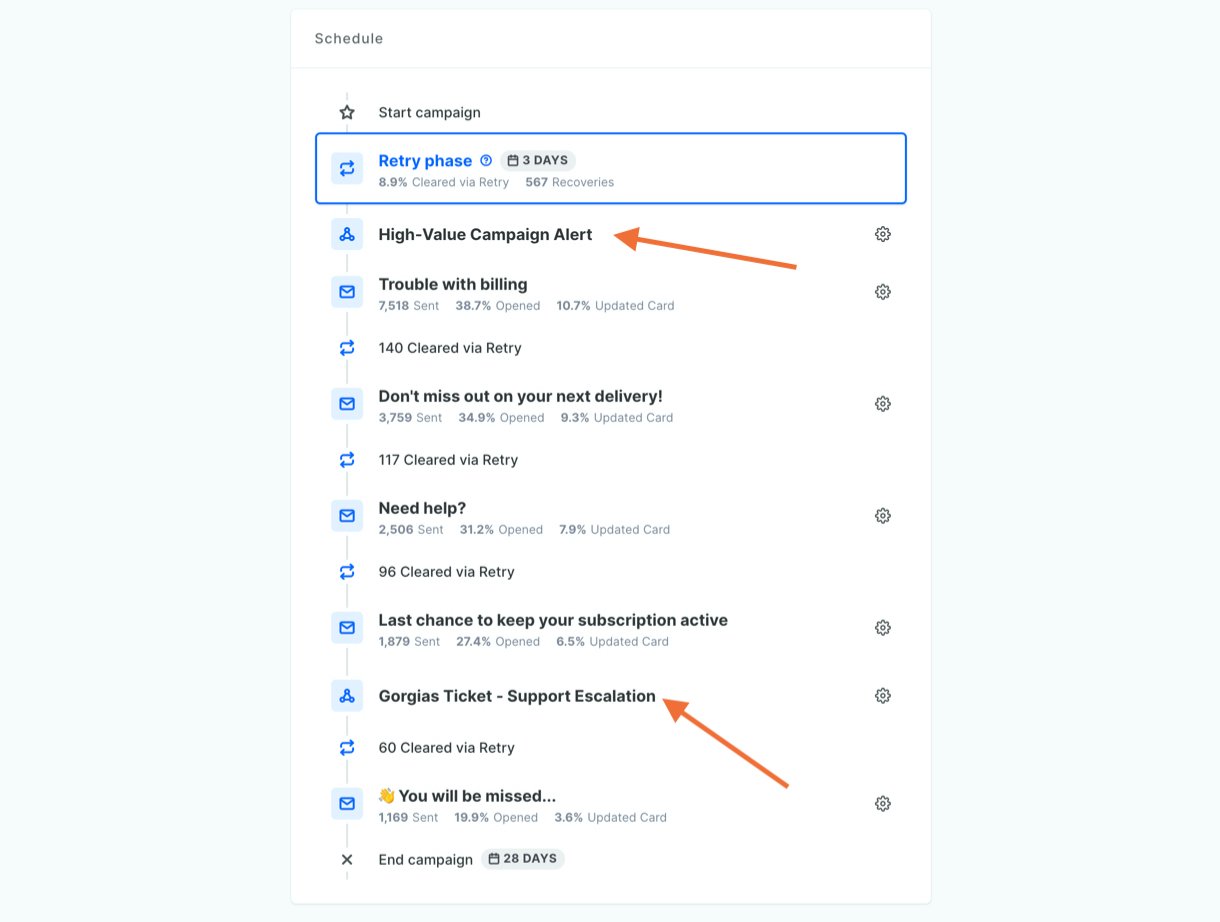In the upper left corner, the word "Schedule" appears in small text. A couple of inches down, there's an image of a star next to the text "Start Campaign," and this area is highlighted with a long blue rectangle labeled "Retry Phase" with an accompanying duration of three days. 

Below this, the text "8.9% cleared via retry" is displayed, followed by "567 recoveries." In black text, it reads "High Value Campaign Alert," highlighted by an orange arrow pointing toward it. To the right, there's a small settings icon resembling a wheel. 

Further down, the text "Trouble with billing" is shown, accompanied by the figures "7,518" (38.7% opened) and "10.7% updated card," with "140 cleared by a retry" underneath. 

Next, the message "Don't miss out on your next delivery!" is displayed with "117 cleared by retry" below it. The phrase "Need Help?" appears, followed by "2,506 sent" and "96 cleared by a retry." The text "Last chance to keep your subscriptions active" is shown alongside the note "Gorgias ticket support escalation," with an arrow pointing toward it. 

Finally, it reads "Cleared by a retry" and concludes with "You will be missed" alongside the note "End Campaign."